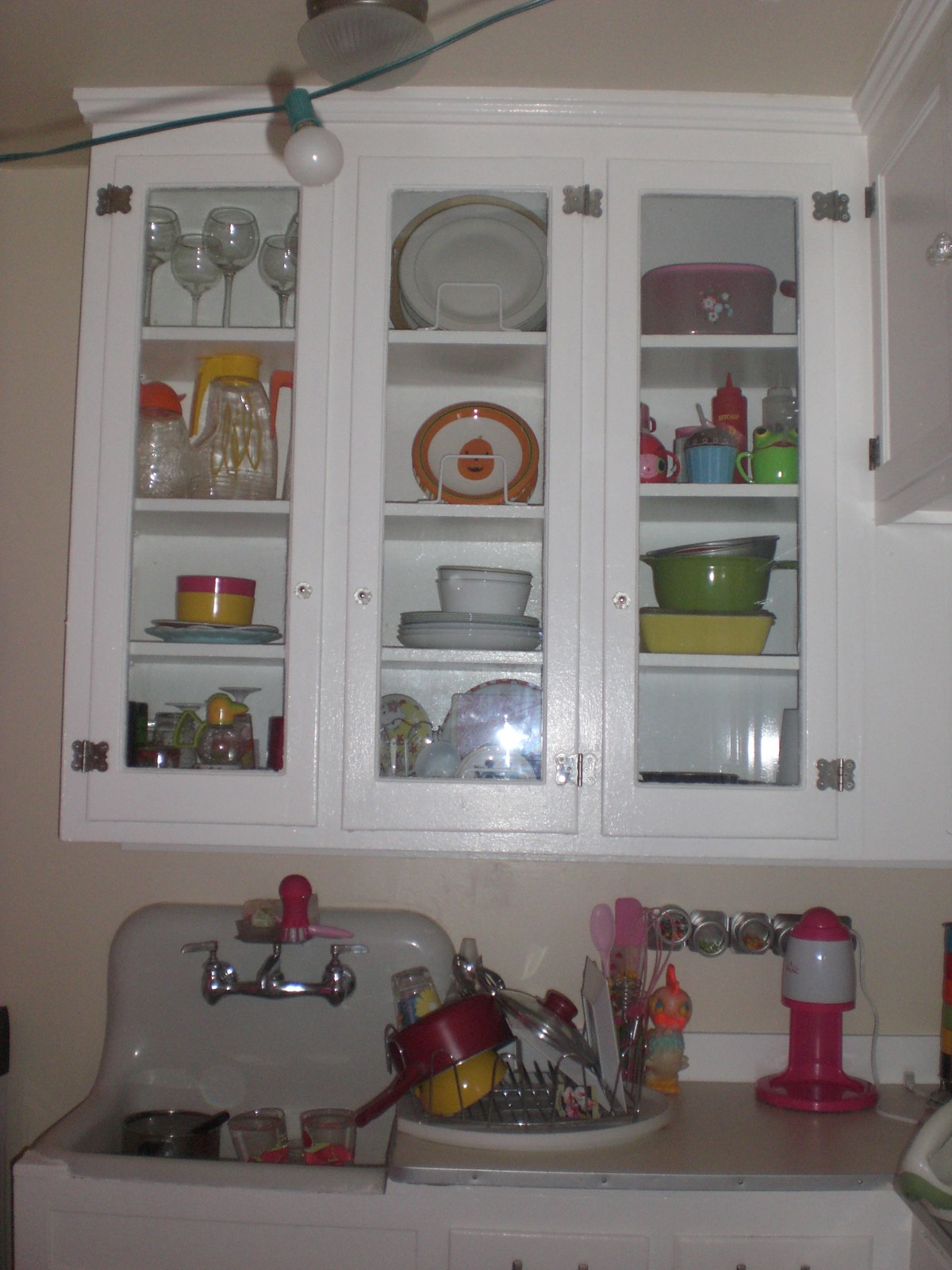In this photograph, a pristine white wall serves as the backdrop for a white cabinet featuring three glass-paneled doors, allowing a clear view of its contents. Inside the cabinet are four shelves meticulously arranged with an assortment of items, including wine glasses, plates, glass bottles, bowls, and cups. Below the cabinet lies a light brown countertop. On this countertop, a red and white object catches the eye next to a small draining board holding various dishes. Among these dishes, there is the lid of a pot, a red pot, and a yellow cup seated underneath. Adjacent to the draining board is a compact white sink with silver taps. Above the tap, a red item stands out, while within the sink, there are two clear cups and a darker object.